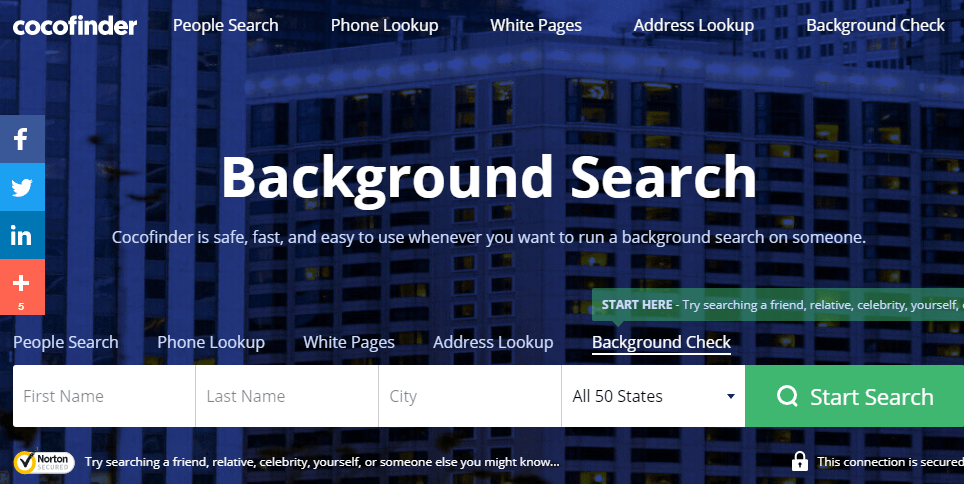The image depicts an advertisement banner on a website called "Cocoa Finder." The banner is designed with a green background and hosts a variety of functional tabs and text elements. 

In the top-left corner, the Cocoa Finder logo is prominently displayed, accompanied by navigation tabs labeled: "People Search," "Phone Lookup," "White Pages," "Address Lookup," and "Background Check." Centrally positioned, large text announces, "Background Search. Cocoa Finder is safe, fast, and easy to use whenever you want to run a background search on someone."

Below this central text, several user interaction elements are arranged. A green backgrounded area with white text reads, "Start here: try searching a friend, relative, celebrity, yourself." Below this, input fields are provided for users to enter the first name, last name, city, and state (with a dropdown menu for all 50 states). Adjacent to these fields is a search button labeled "Start Search."

The footer section of the banner reiterates the service's security and ease of use with a note: "Not unsecured, try searching a friend, relative, celebrity, yourself, or someone else you might know, this collection is secured." 

In the background of the image, a slightly blue-tinted night scene is depicted, featuring a massive building with numerous windows. To the left side of the banner, social media icons for Facebook, Twitter, and LinkedIn are visible, along with an additional icon that reveals further sharing options upon interaction.